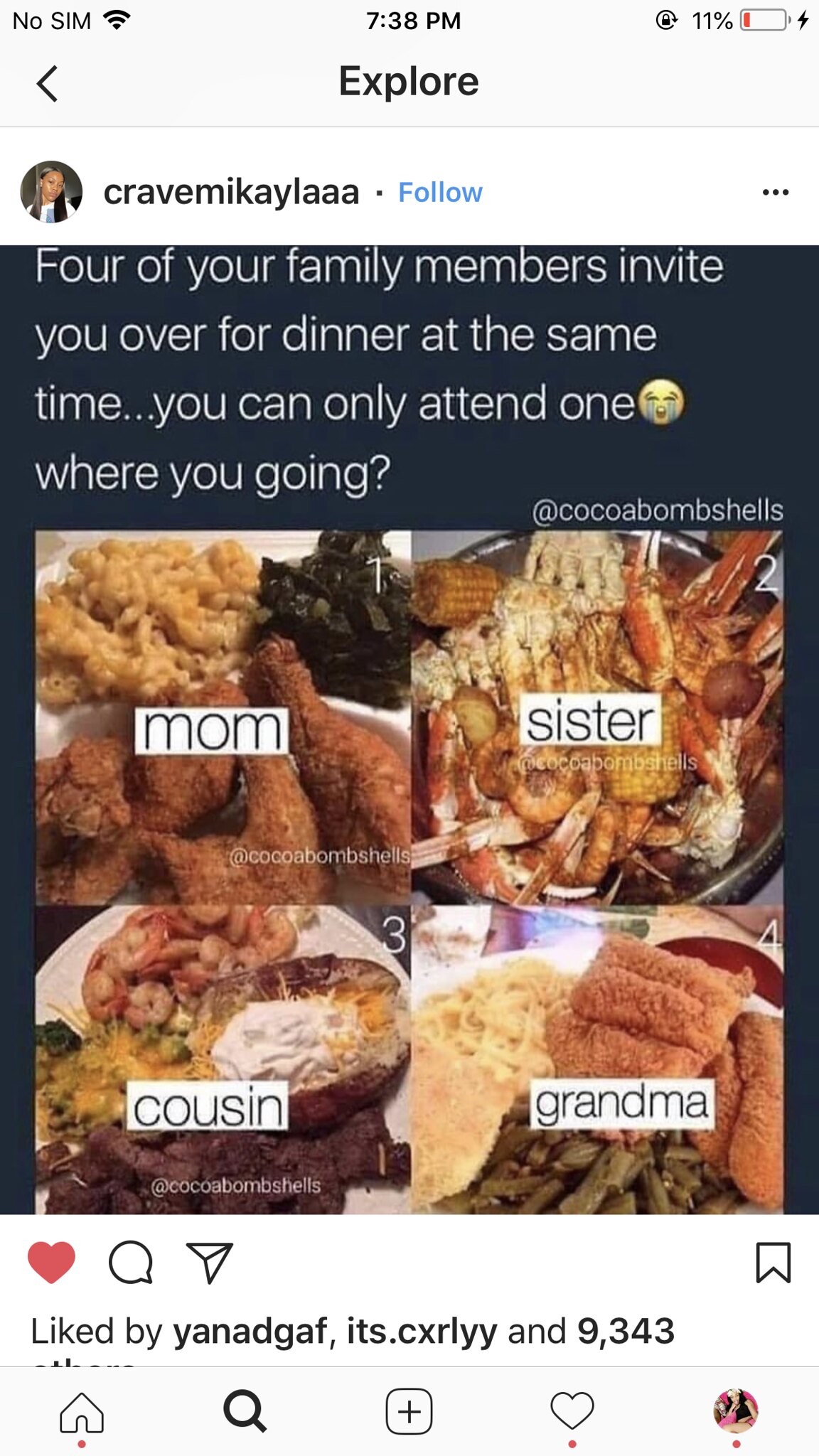This color photo is a screenshot of an Instagram post from the Explore page, shared by user @CraveMikayla. Visible on a phone screen at 7:38 PM with an 11% battery indicator and a "no SIM card" status, the lively meme at its center proposes a playful dilemma: "Four of your family members invite you over for dinner at the same time. You can only attend one. 😢 Where are you going?" The black background sets off four delectable meal options, each associated with a different family member. In the top left, Mom offers crispy fried chicken, creamy mac and cheese, and savory collard greens. Adjacent to this, Sister tempts with a bountiful seafood boil featuring lobsters and corn on the cob. Below, the Cousin entices you with a fully-loaded baked potato, juicy barbecue meat, and plump shrimp. Finally, Grandma, in the bottom right, serves up comforting chicken-fried steak, mashed potatoes, and green beans. The meme, tagged @CocoBombshells, is immensely popular, evidenced by likes from users like Yanad Gaff and It's Curly, and 9,343 others. The top-center of the image shows the word "EXPLORE," above an avatar and username.